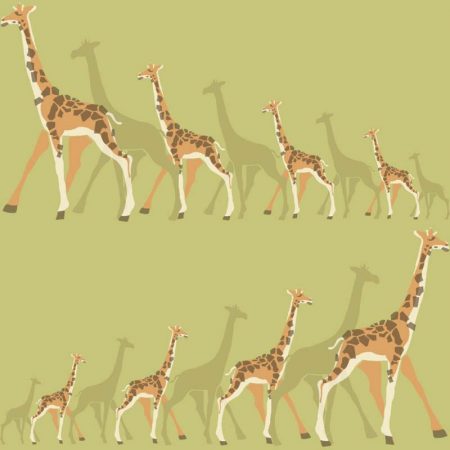This image features eight digitally created giraffes set against a light, beige-green background. The giraffes are arranged in two rows: the bottom row has four giraffes walking from left to right, and the top row features four giraffes walking from right to left. In the bottom row, the giraffes are ordered from smallest to largest, while in the top row, they are organized from largest to smallest, creating a mirror image effect. Each giraffe has a tan-orange body with dark brown spots and white or cream-colored accents around their legs and ears. Between each giraffe is a shadow matching the size and direction of the respective giraffe. This tableau, devoid of any text and resembling a line drawing or clip art, presents a gentle, somewhat muted visual experience.